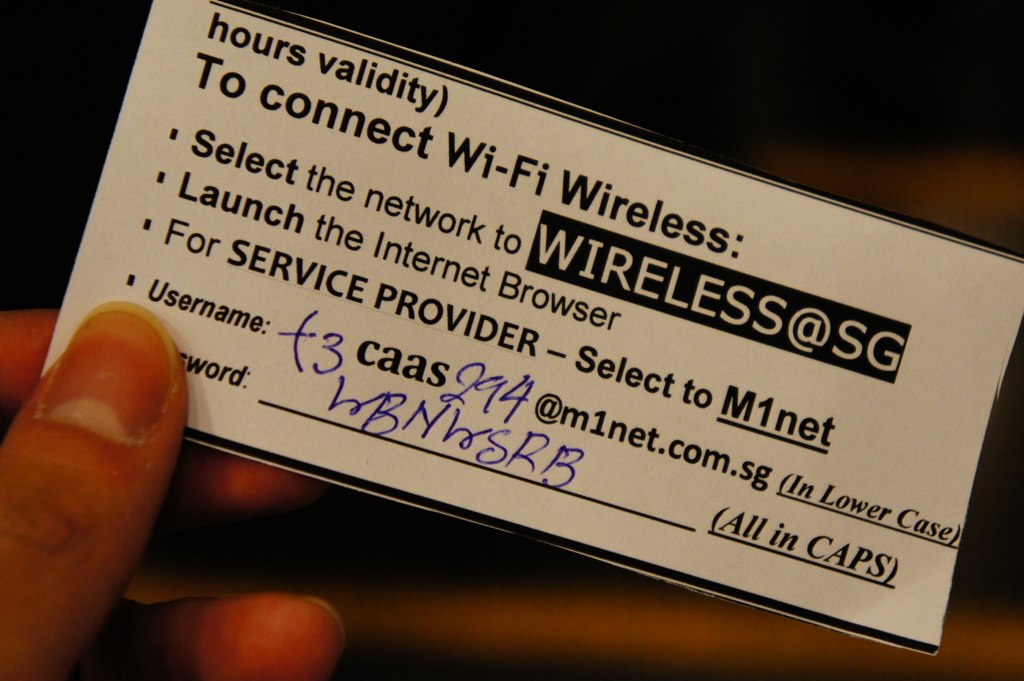In the image, a person is holding a white, rectangular card using their left hand, with their thumb and part of their other fingers visible toward the right edge of the image. The background is dark, highlighting the card in the person's hand. The card contains instructions for connecting to a Wi-Fi network. At the top, it reads "Hours Validity" followed by "To connect Wi-Fi wireless" in black letters. Below this, there are several bullet points. The first bullet point, in bold black text, says "Select," followed by "the network to wireless at SG," where "wireless at SG" is enclosed in a black rectangle with white text and an at symbol (@). The next bullet point, also in bold black text, reads "Launch internet browser." The subsequent point says "For service provider," in standard black text, followed by "select to M1net," where "M1net" is written continuously. Under these instructions, the card lists a username: "3caas294@m1net.com.sg" (with the digits "3" and "294" in blue ink) and specifies "in lowercase" in parentheses. The password, partially obscured by the person's thumb, appears to include "WBNWSRB" with "all in caps" noted in parentheses. The card has minimal decoration with a slight tilt so that the left side is angled towards the upper left of the image, and the right side is angled towards the bottom right, giving it an instructional and utilitarian appearance related to logging into a router or Wi-Fi network.